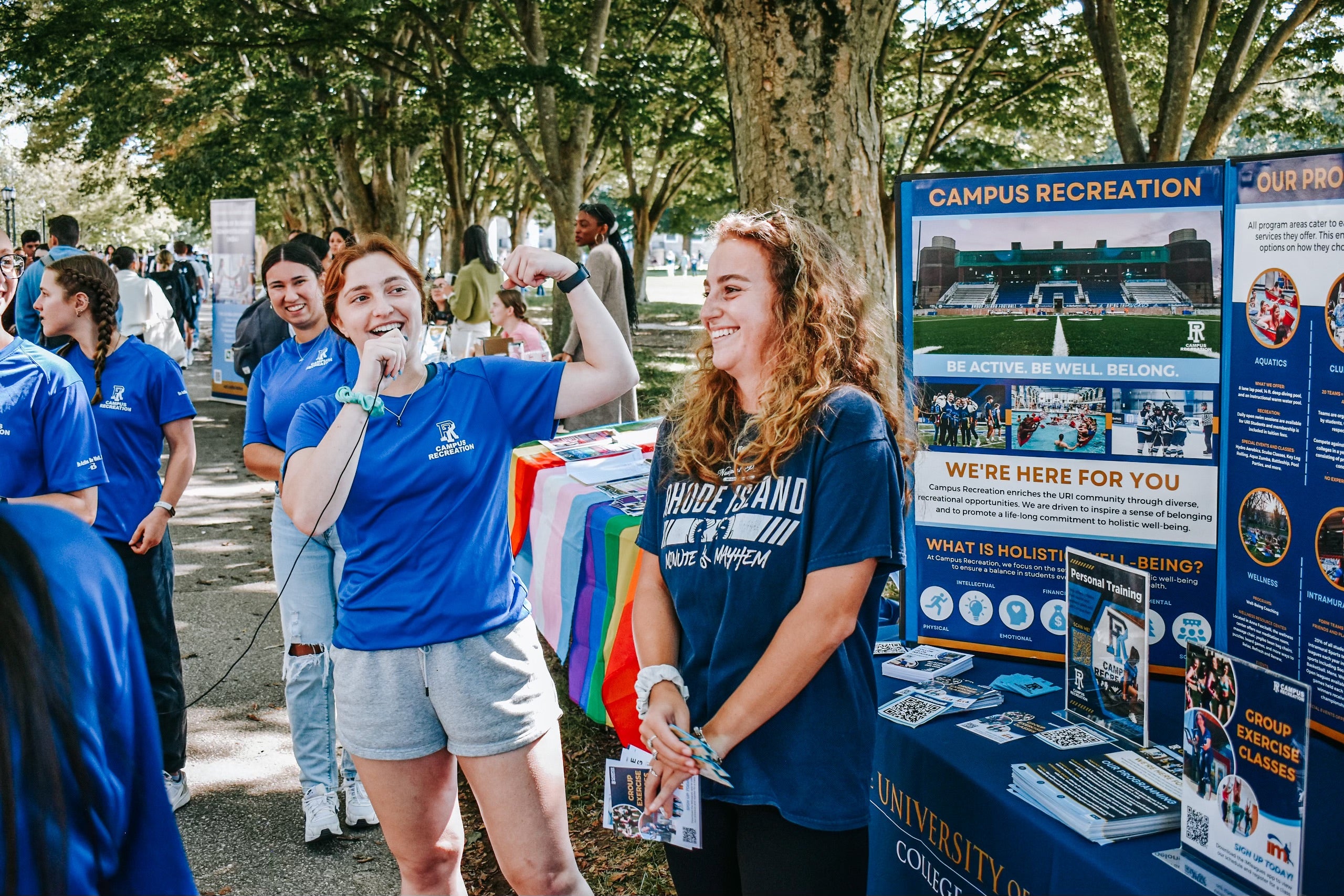This photograph depicts an enthusiastic and welcoming event at the University of Rhode Island, likely aimed at welcoming freshman students or recruiting new members for campus activities. Central to the image are two young women standing near a table adorned with large posters on a blue background that prominently feature messages such as "Campus Recreation, We're Here for You" and "Be Active, Be Well, Belong." One of the women, dressed in a blue t-shirt and gray shorts, holds a microphone and is energetically speaking, her arm raised in a gesture of confidence. She is looking at her companion, who is smiling broadly and holding informational brochures, while wearing a shirt emblazoned with "Rhode Island." Both women's expressions exude joy and community spirit. Surrounding them are numerous students, suggesting a lively and engaging atmosphere. The event is set outdoors under a canopy of leafy trees, indicating it takes place during spring or summer. The vibrant colors of blue, dark blue, light blue, black, red, yellow, green, white, brown, and beige further add to the image's lively and inviting ambiance. In the backdrop, additional students mill about, and the overall scene highlights a sense of belonging and commitment to holistic well-being promoted by the university's recreational activities.